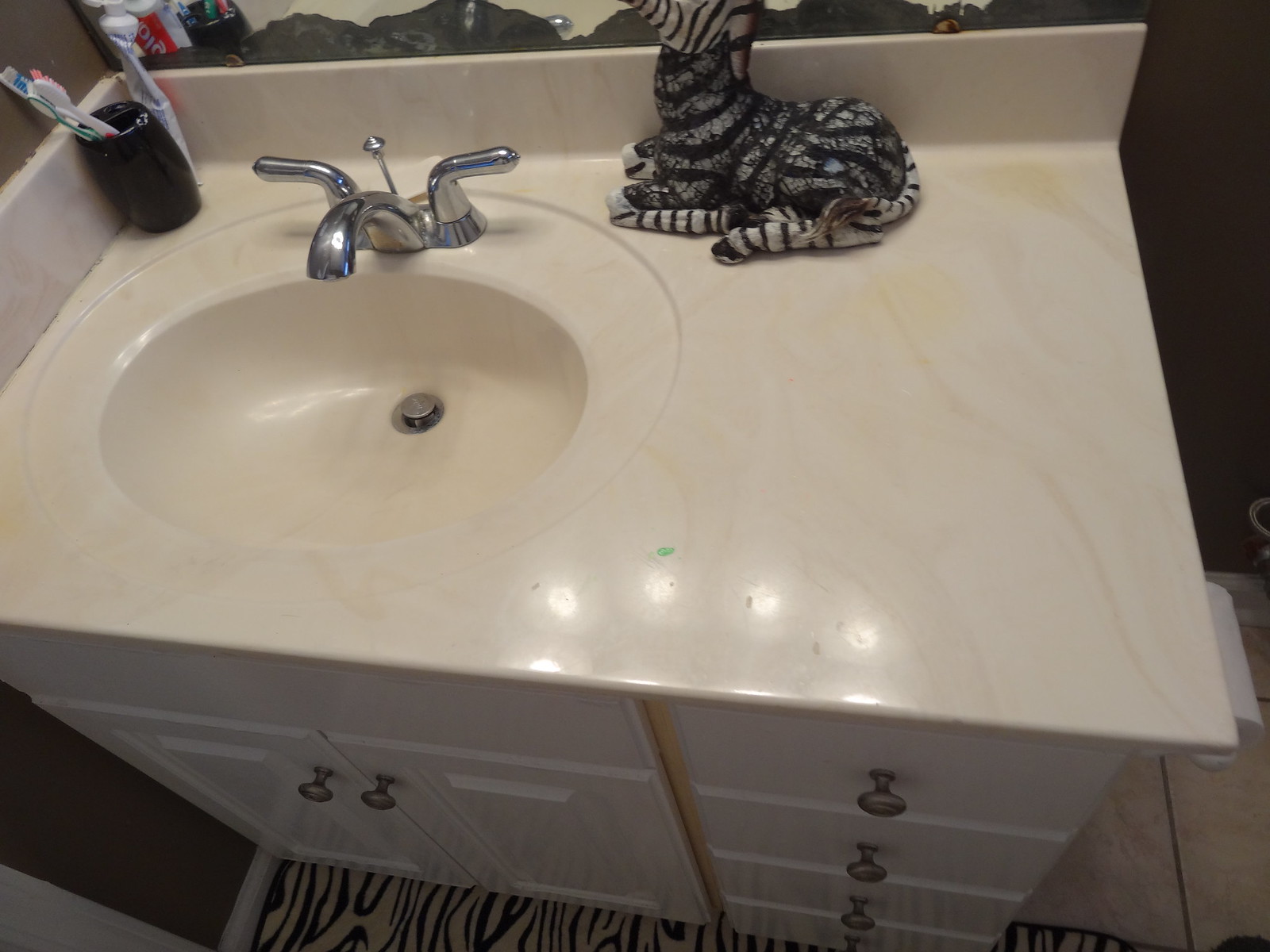The image captures a detailed view of a bathroom counter. The grayish-brown corner of the wall meets a mirror mounted above the sink. A zebra print carpet adds a wild touch to the floor in front of the sink vanity area, while the white tiles with gray grout form the backdrop. To the right, a white roll of toilet paper is visible along with a small section of one of the toilet’s access pipes. 

The vanity itself is an elegant white cream marble, featuring a continuous smooth surface that extends into the sink basin. The sink is equipped with both hot and cold water taps and has a stopper in the middle. Atop the sink, there is a black toothbrush holder with three toothbrushes lined up closely inside. Behind this, a tube of white Colgate toothpaste with its distinctive red logo can be seen.

In the right corner of the counter space, a tiny green speck stands out, presumably toothpaste or possibly nail polish. Adding a decorative touch, at the far end of the counter, there is a ceramic figure of a black and white striped cat, about the size of a rectangular Kleenex box. 

The base of the sink features cabinets and drawers accented with bronze knobs. This image effectively showcases a section of a bathroom sink area, combining functional and decorative elements in a seamless manner.